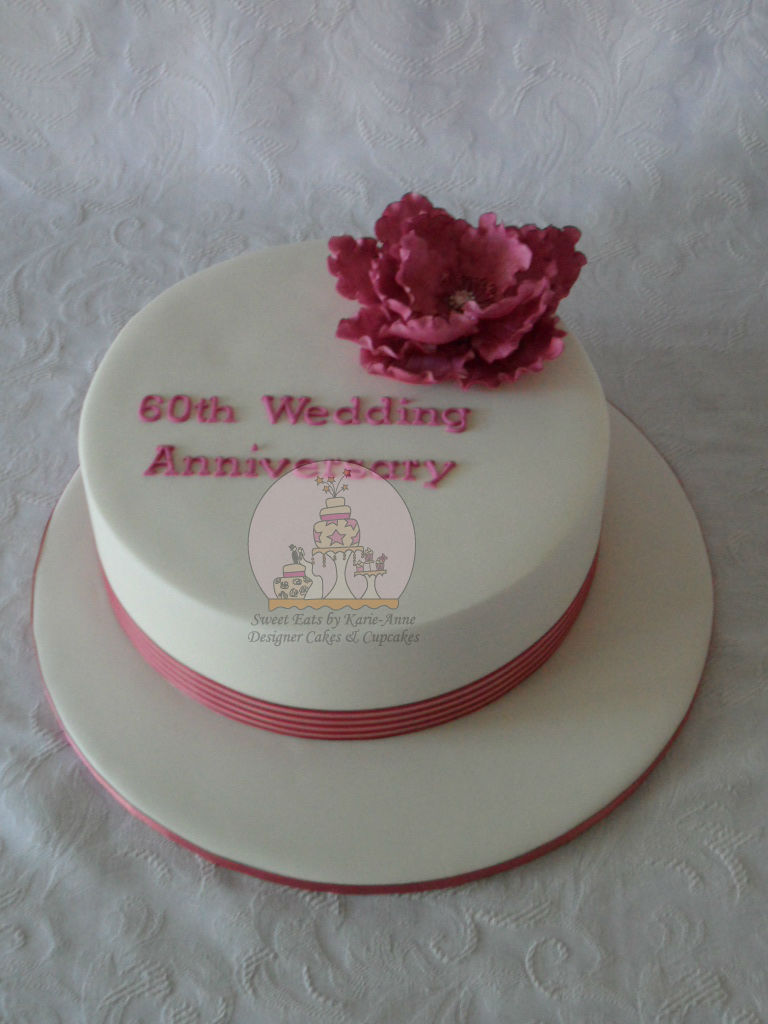The photograph captures an elegant cake designed to resemble a stylish top hat, celebrating a 60th wedding anniversary. The cake is meticulously crafted with a blend of white and beige tones, accented by red trims at the base and the top of the two-tiered structure. The top tier is adorned with a detailed red lettering that reads "60th Wedding Anniversary." Complementing the design is a delicate pink rose positioned at the top right of the cake, likely crafted from sugar. A notable watermark at the center of the image reveals a circular, snow globe-like logo depicting a central white cake with red stars, flanked by two smaller cakes, all underlined with the text "Sweet Eats by Kate - Designer Cakes and Cupcakes" in small black font. This exquisite cake is set against a white tablecloth subtly patterned with white floral designs, adding to the overall sophisticated aesthetic.